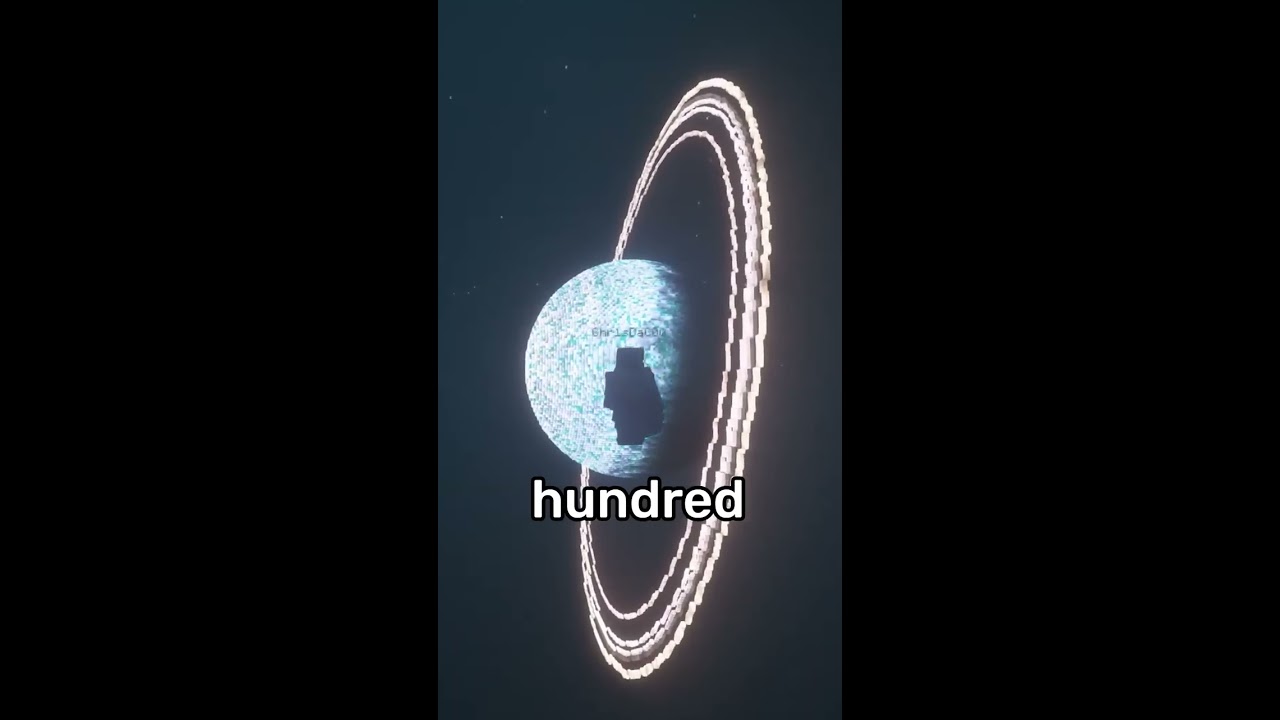The image in question is a minimalist, portrait-style computer graphic featuring a turquoise blue planet set against a dark grey background. The planet, reminiscent of Uranus or a rotated Saturn, has distinctive, jagged, pixelated rings encircling it vertically rather than the conventional horizontal alignment seen in natural celestial bodies. A navy blue marking on the planet suggests a redacted-like appearance, adding to its unique look. Centered towards the bottom of the image is the white text "100" spelled out as H-U-N-D-R-E-D. The overall resolution appears pixelated and somewhat old-fashioned. The portrait image is presented within a larger landscape frame, with thick black panels on both the left and right sides, enhancing the contrast and drawing focus directly to the central planetary figure.